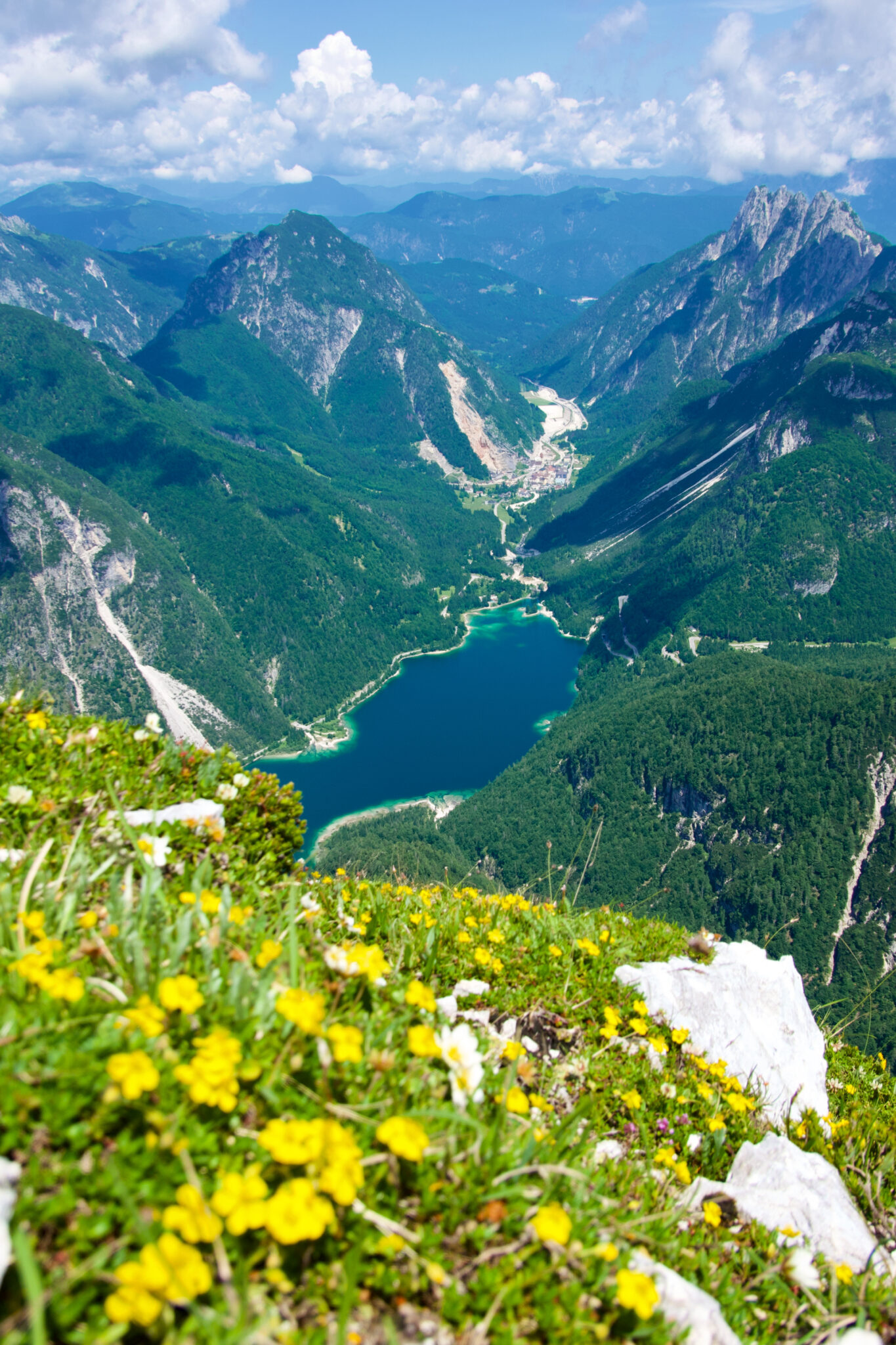The photograph captures a stunning outdoor landscape, taken from atop a mountain or hill, overlooking a vibrant valley. A large body of water, resembling a fjord or clear blue lake, stretches below, with greener water closer to the shoreline and darker blue hues further out. The shoreline features clear, inviting beaches. Tall, powerful green mountains rise majestically on either side of the valley, covered in lush vegetation, evidence of springtime. In the far-off distance nestles a small town, with tiny buildings and roadways, surrounded by the towering mountains. The foreground is rich with low-lying plants, including blooming yellow and pink flowers, interspersed with whitish-gray rock outcroppings and dark green grassy areas. Signs of erosion and a dry riverbed indicate past water flow into the fjord. Overhead, the sky is mostly clear with scattered puffy clouds, adding to the breathtaking vista of mountains, water, and vibrant spring growth.